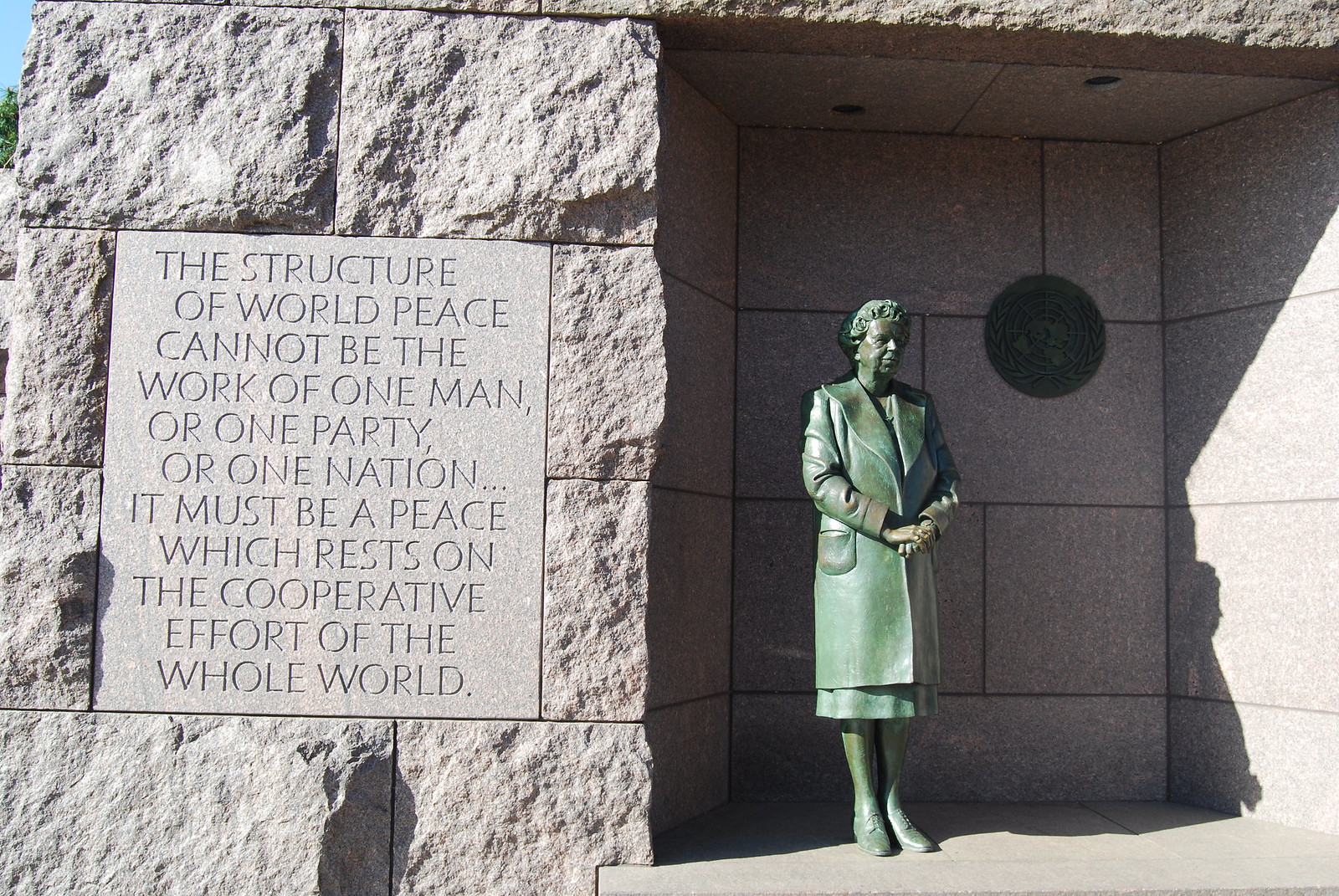The photograph captures a significant monument resembling a mausoleum. Dominating the right side of the image is a statue of a woman, meticulously crafted in a green hue, encapsulating the fashion of the 1950s with her distinct hairstyle, shoes, and a long coat. She bears a resemblance to a presidential figure's wife. To the left, there's a prominent stone sign etched with a profound message: "The structure of world peace cannot be the work of one man or one party or one nation. It must be a peace which rests on the cooperative effort of the whole world." The structure is framed under a concrete ceiling with a sliver of blue sky visible above, contrasting the gray stone of the monument. The photograph, likely taken in a museum setting, showcases the statue's solemn presence and the powerful inscription that accompanies it, emphasizing a universal call for collaborative peace.